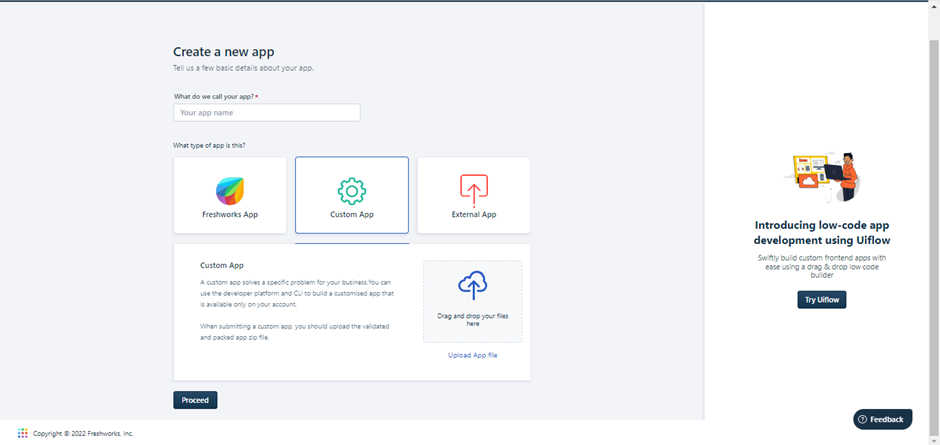In this image, we see a detailed interface for creating a new app. The page is presented with a light gray background, making the interactive elements stand out on the user interface.

On the left side of the page, there is a prominent section titled "Create an App." This section provides basic instructions and fields for initiating the creation of a new application. The interface asks, "What do we call your app?" and provides a text bar where users can input the app's name. 

Directly below the text bar, there is a menu with options representing different types of apps that can be created. The options include:

1. **Freshworks App**: Illustrated with a colorful leaf icon.
2. **Custom App**: Represented by a settings gear icon.
3. **External App**: Marked by an upload icon.

In this specific instance, the "Custom App" option is selected. A description of what a Custom App entails is provided in two paragraphs beneath the selection menu. Adjacent to this description is a drag-and-drop area where users can upload app files, labeled "Upload App Files."

At the bottom of this section, a small blue button labeled "Proceed" allows users to move forward with the app creation process.

To the right side of the page, there is another section featuring a drawing of a young man holding a laptop. This drawing is positioned next to an illustration of a desktop computer on a desk, with a cloud icon above it. This section is introducing "Local App Development Using UI Flow," giving users a brief overview of this feature. Below this introductory text, there is a box with an option to "Try UI Flow."

At the very bottom of this right section, there is a feedback link, inviting users to provide their input on the interface or process.

Overall, the image portrays a well-organized and user-friendly interface designed to guide users through the initial steps of creating a new app, offering various options and supportive illustrations to facilitate the process.